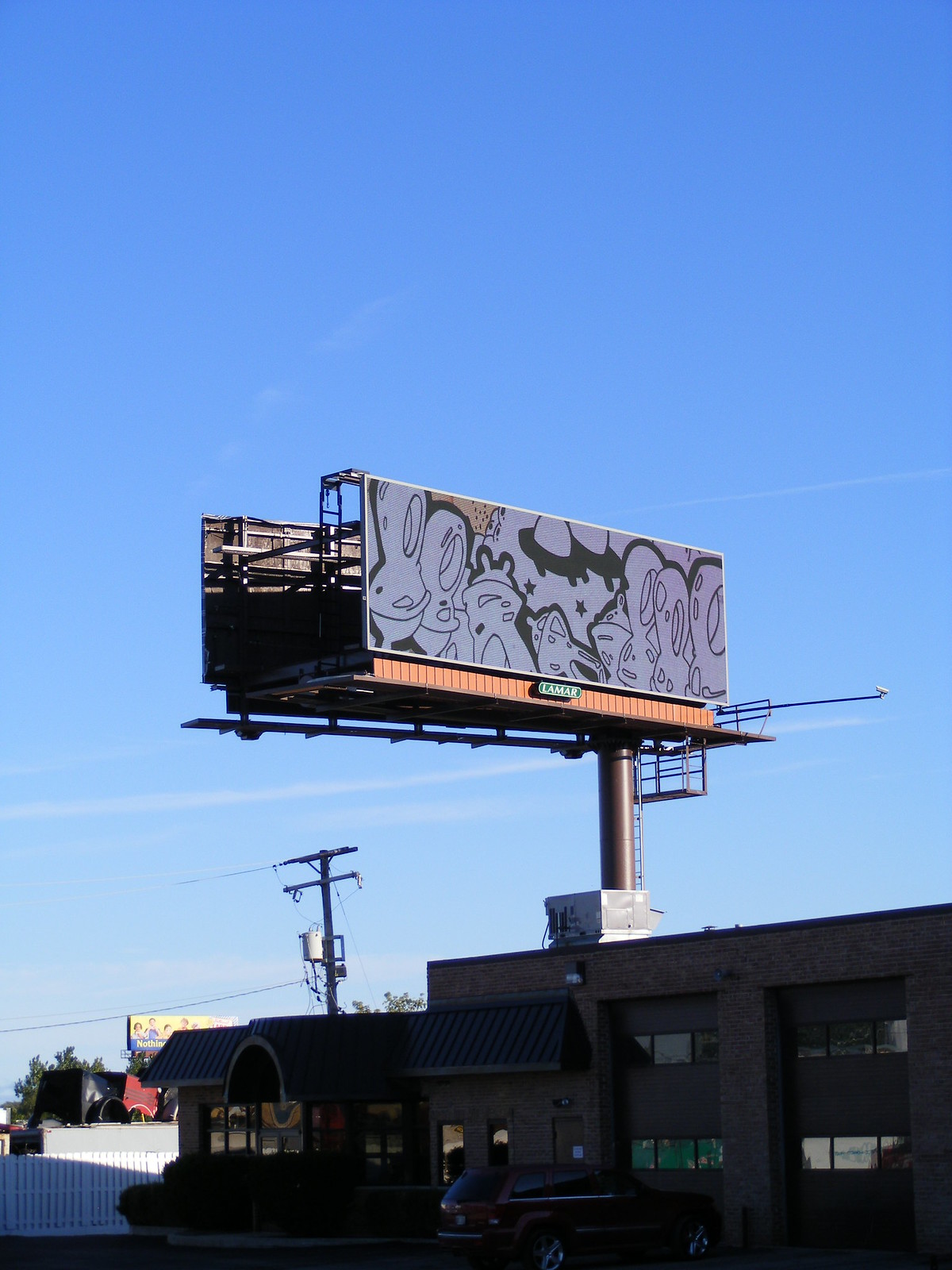In the image, a large billboard is prominently displayed behind a shorter office building. The billboard, positioned towards the top, features an abstract black and white design with hints of peach and tan colors, giving it an almost whimsical portrayal of what appears to be rabbits and aliens, though the figures are not clearly defined. At the bottom of the billboard, there is a green section bearing the name "Lamar." The office building in the foreground is quite modest in height compared to the towering billboard. Parked in front of the office building is a maroon SUV, resembling a van. The scene is set under a blue sky, visible in the upper left corner of the image.